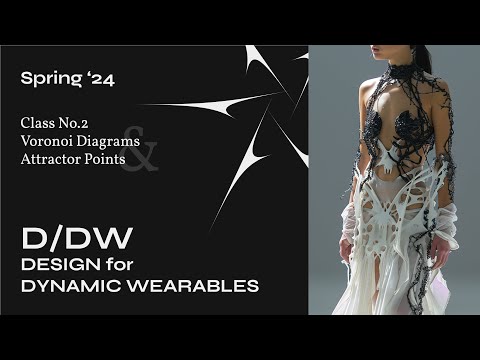The image is an advertisement for a futuristic women's fashion line titled "Spring 24, Class Number Two: Voronoi Diagrams Attractor Points," designed by DW for Dynamic Wearables. Set against a stark black background, the left side of the image features the descriptive text along with a distinctive emblem that resembles a throwing star with pointed, narrow tips. On the right side, a model showcases a highly avant-garde dress composed primarily of black strings that intricately cover her upper body, resembling a bra and ropes around her neck extending to her arms. The dress transitions into white, flowing fabric around her lower legs and wrists, characterized by a Swiss cheese-like pattern with multiple holes, emphasizing minimalistic and dynamic design.